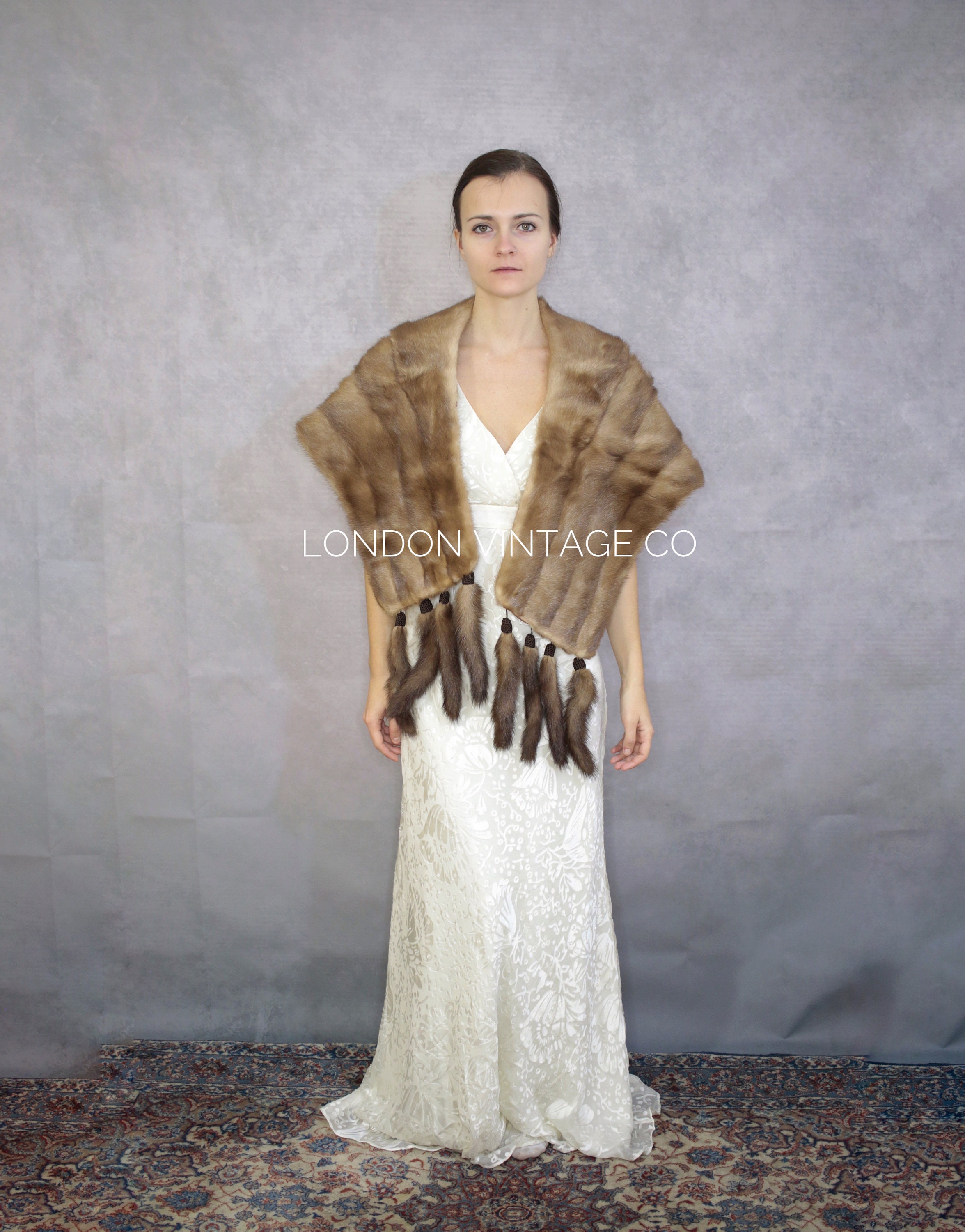In this image, a woman stands poised, looking directly into the camera, with the words "London Vintage Co. CEO Company" written in white lettering. The background is a basic grey wall, creating a neutral backdrop for the scene. She stands on an oriental rug that features a vintage design with blue, brown, tan, and hints of red, adding more color to the composition.

Her hair, which is dark brown or black, is pulled back and presumably tied into a bun, giving it a very sleek appearance. Although her facial expression is neutral, it imparts a somewhat somber or serious tone. She is modeling an elegant, long white dress that has a subtle floral pattern, with the flowers being in lighter shades of white.

Draped over her shoulders is a large fur scarf, which extends down to her waist. This scarf, possibly made from animal fur, is predominantly brown with black-tipped tails hanging from it, adding texture and depth to her outfit. The detailed and luxurious fur piece is stitched together in sections and features four long projections on each end that resemble rabbit tails. The overall aesthetic combines elements of vintage charm and high-fashion sophistication.